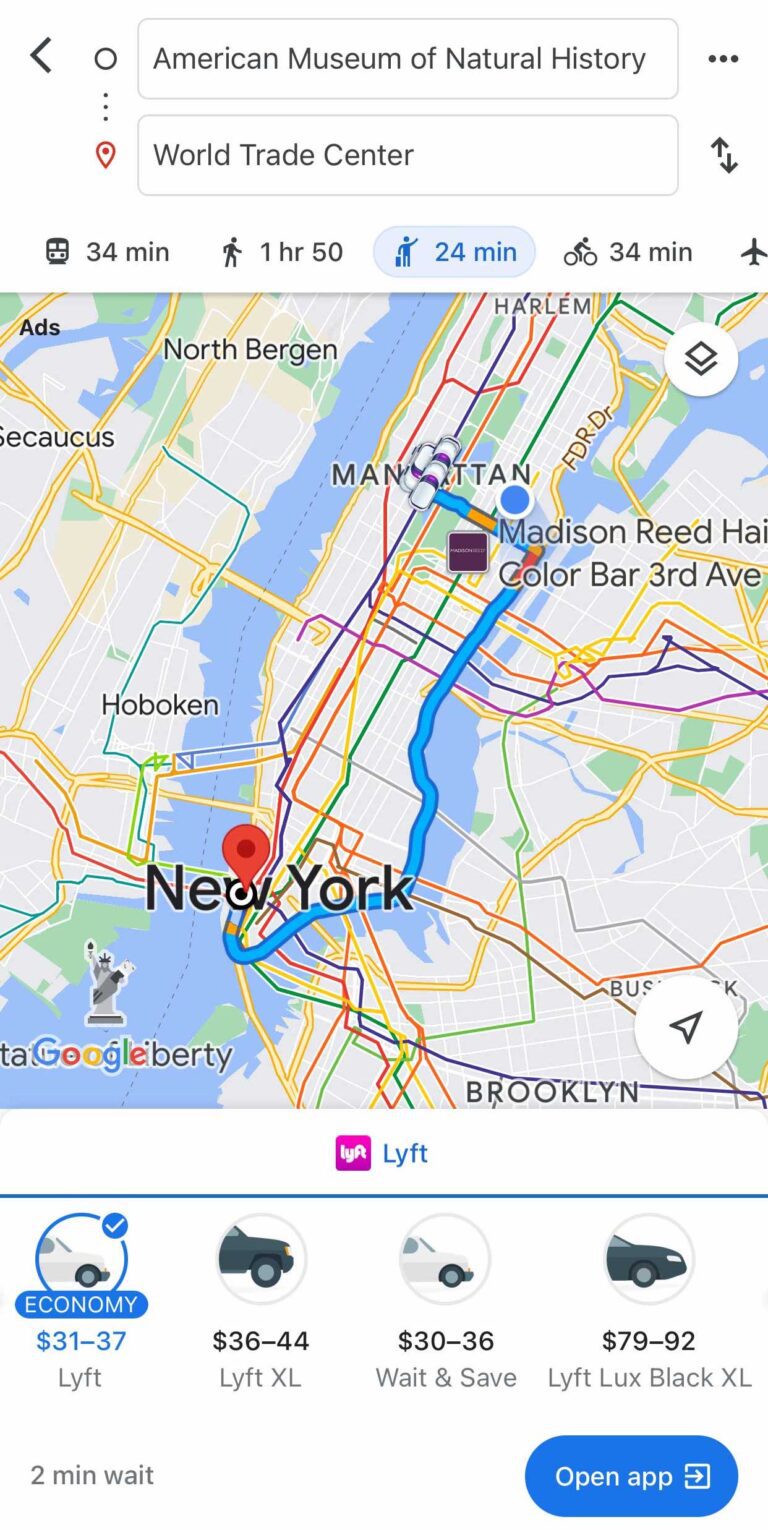The image is a detailed screenshot of a navigation-oriented app, prominently featuring a map interface. At the top of the screen, a Google Maps layout displays two location bars: the starting point, "American Museum of Natural History," and the destination, "World Trade Center." On the top left of the interface is a back icon, while the top right shows a three dots icon for additional options, beneath which lies a swap icon for reversing the route.

Immediately below the location bars is a white section containing five transportation options: a bus icon labeled "34 minutes," a walking icon labeled "1 hour 50 minutes," a man with a briefcase icon labeled "24 minutes," a cycling icon labeled "34 minutes," and an airplane icon. The "man with a briefcase" icon, signifying a fast trip of 24 minutes, is highlighted in blue, indicating the selected mode of transportation.

Central in the display is an expansive map, showcasing various elements such as highways, green areas, water bodies, and potential transit lines. The lower left corner of the map features the Google logo, accompanied by an icon of the Statue of Liberty. A prominent red pinpoint marks "New York," while a blue circle in the top right indicates the user's current location somewhere in the city, amidst several white vehicle icons symbolizing available transport means.

At the screen's bottom is a horizontal white bar, listing multiple vehicles along with their corresponding dollar rates, all underpinned by the Lyft logo, suggesting ride-sharing options for the user.